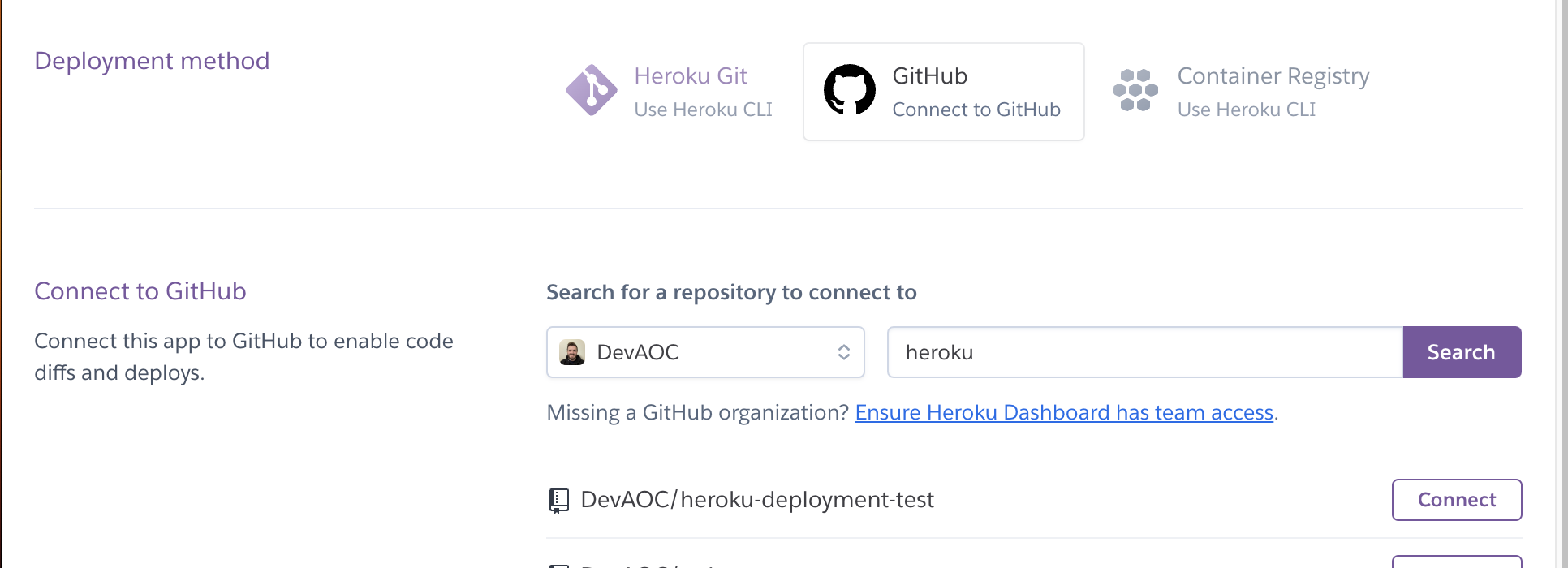This image is a screenshot from a website with a white background, featuring a configuration menu for deployment methods. The interface appears to be related to Heroku, not GitHub, although it includes options for GitHub integration. At the upper left corner, there's a label titled "Deployment method." 

From the center extending to the right, there are three sections:
1. **Heroku Git**: Indicated as “Heroku Git” with further instructions stating "Use Heroku CLI."
2. **GitHub**: Highlighted in the middle with the GitHub logo—a small circle featuring a stylized white drawing of an animal, possibly a cat or mouse, with ears on either side. Beneath the logo, it says "Connect to GitHub."
3. **Container Registry**: Positioned on the right, stating "Use Heroku CLI" for further details.

Beneath these sections, specifically on the left side, there's additional text explaining the functionality: "Connect this app to GitHub to enable code diffs and deployments." This reinforces that the menu is providing options to connect the app to GitHub, rather than it being a GitHub interface itself.